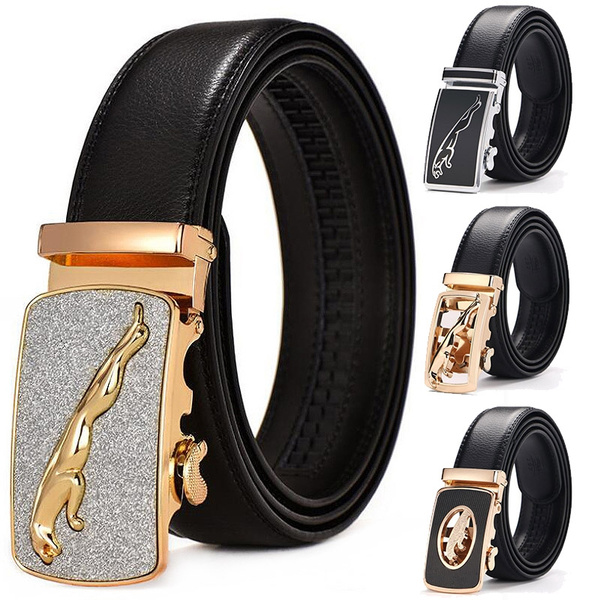This photograph, likely from a product listing or advertisement, showcases four black leather belts rolled up and displayed against a stark white background. The leftmost belt is prominently larger than the others, featuring a gold buckle with a sparkly silver inlay and a golden leaping jaguar at its center. To its right, three smaller belts are vertically aligned, each with a unique metallic buckle design. The top belt sports a silver buckle with a black background, highlighted by a silver jaguar with black details. The middle belt has a brass buckle adorned with abstract geometric patterns, which appear to blend red and white colors. The bottom belt features a brass buckle with a black vertical inset, housing an indiscernible golden icon that may also represent a jaguar. The belts, angled at three-quarters facing left, emphasize the variety of intricate buckle designs available.